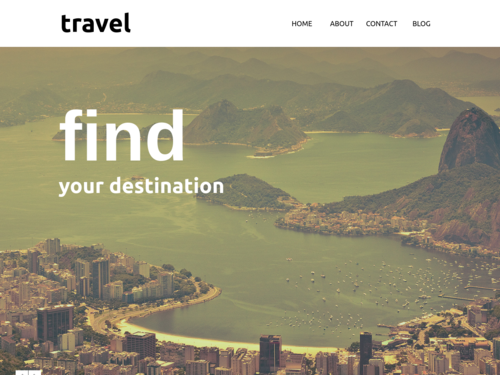The image depicts a cluster of islands, with several of them featuring mountainous terrains. The largest island, centrally positioned, hosts a bustling cityscape characterized by numerous tall buildings. The atmosphere appears foggy, with the sky enveloped in shades of gray, contributing to a moody and misty ambiance. Prominently, the words "Find Your Destination" are displayed in bold white font, significantly larger than the rest of the text. At the top left corner, the word "Travel" is visible, while the top right corner features navigational links labeled "Home," "About," "Contact," and "Blog."